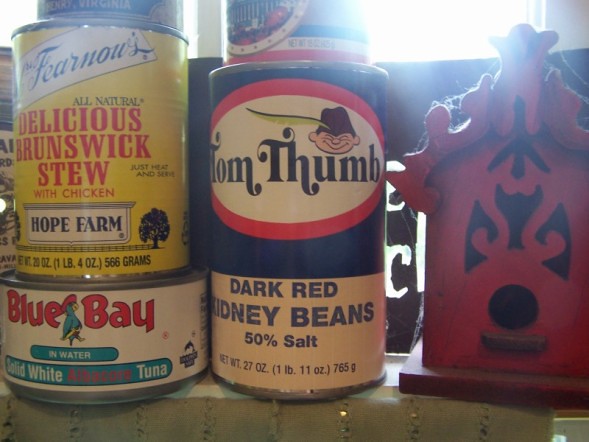The photo depicts an indoor scene illuminated by sunlight streaming through a window, casting a warm glow on a brick ledge where an assortment of vintage food cans are displayed. The foreground features an old-fashioned can of "Tom Thumb" dark red kidney beans, adorned with a blue background and a striking red circle with white text. The label showcases an elf-like character and mentions that the beans contain 50% salt. Adjacent to it is a can of Brunswick stew with chicken, dressed in a yellow label that reads "Hope Farm," although the brand name is slightly obscure due to a quirky font and slight blurriness. Beneath the stew can, a Blue Bay tuna can is partially visible, contributing to the nostalgic ambiance of the arrangement.